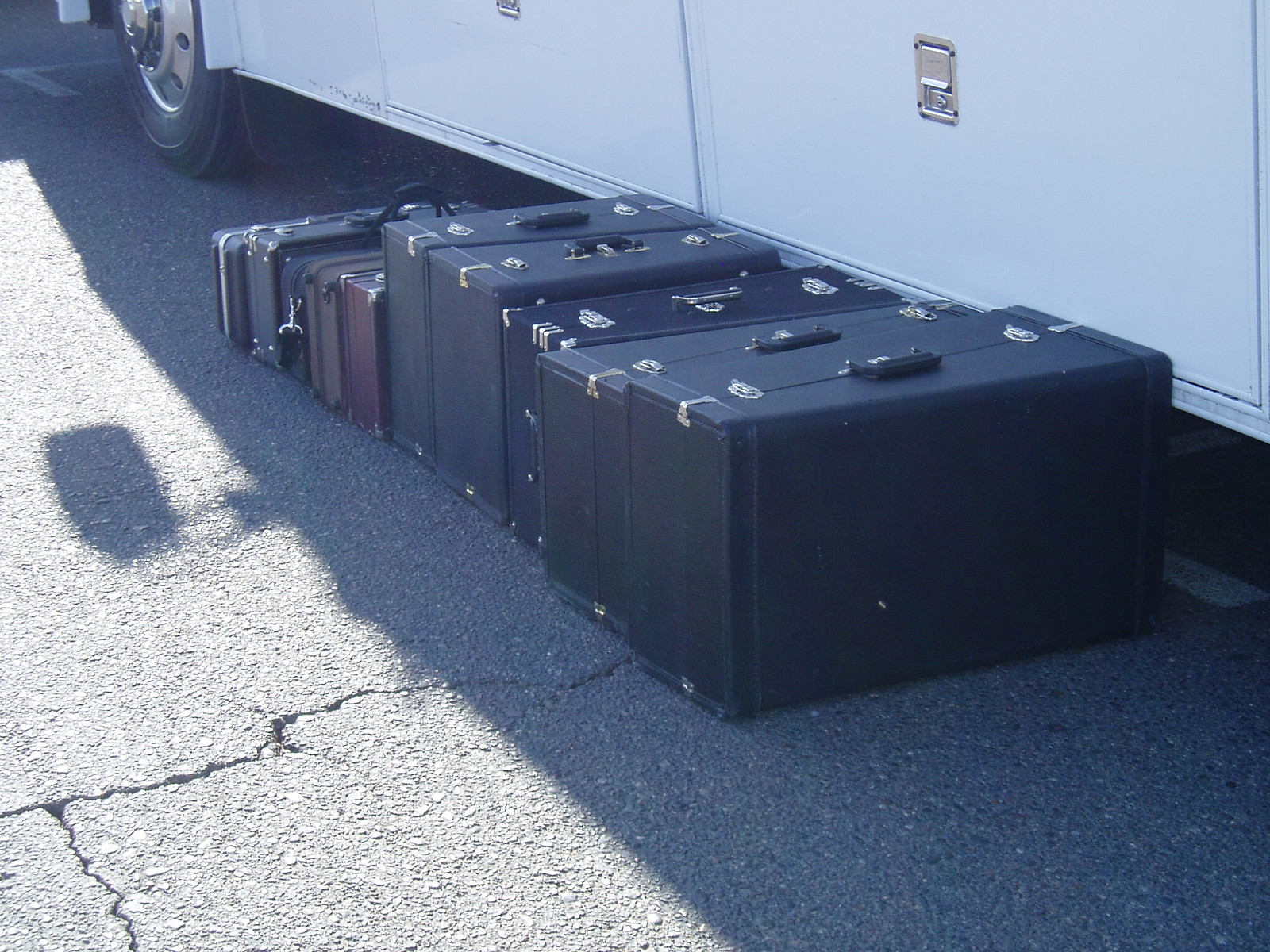The photograph captures a collection of twelve rectangular suitcases, placed on cracked grey asphalt near the luggage compartments of a passenger charter bus. The majority of the suitcases are black with silver locking clasps, and they vary in size, arranged from smaller ones on the top left to larger ones on the bottom right. Among the black cases, there is a distinct brown suitcase on the top left and a burgundy one further to the far end. Overhead, parts of the bus are visible, including silver handles and a white door, as well as a wheel in the top left corner. A black weight and a subtle reflection of a mirror add additional details to the left side of the image.